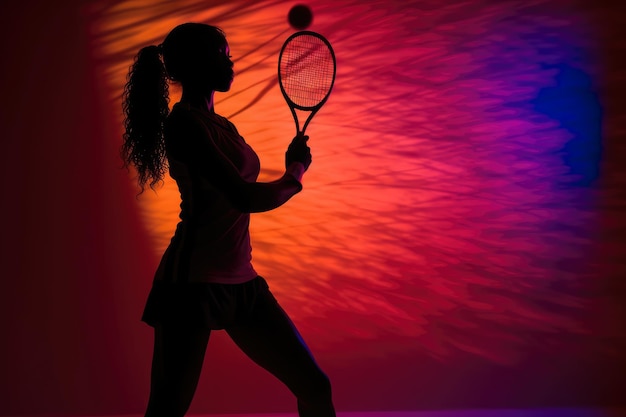In the vividly colorful image, the silhouette of a woman playing tennis commands the center stage. She appears to be a black woman with an athletic build, characterized by her long, curly ponytail that streams from the middle of the back of her head. She is dressed in a classic tennis outfit, including a shirt and a short skirt. The racket, held in her right hand, is poised vertically with a blurry tennis ball hovering just above it, hinting at her recent swing.

The background is a mesmerizing ombre of colors, transitioning smoothly from deep red on the left to bright orange and then to shades of magenta, raspberry, purple, and finally blue towards the right. This vivid backdrop also includes various swirling patterns and lines depicting the motion of her racket, giving the scene a dynamic and almost surreal quality. The multicolored hues—encompassing reds, pinks, oranges, and blues—also reflect off her clothing, further enhancing the dreamlike atmosphere of the image.